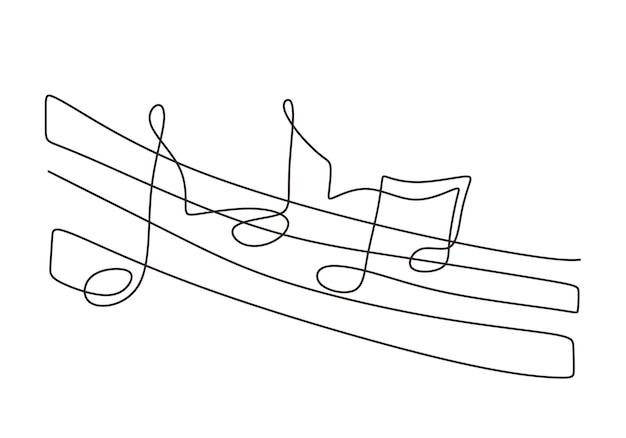This image is a whimsical, almost chaotic representation of musical notes drawn with a single continuous line. The line starts on the right side of the white background, approximately in the middle, and moves diagonally to the left, almost reaching the edge of the page. It then shifts down about an inch, crosses back to the right, and drops about another inch before curling into a loop and forming the first music note. The line emerges from this note and moves left to create the second note, continuing leftward to form a third note. From here, it descends and curves leftward, forming a curly cue right at the edge of the page. The line then ascends about an inch, traverses back to the right, ascends again, and crosses left before finally trailing off the page. The entire drawing gives an impression of squiggly, erratic lines, mimicking the effect of an Etch-a-Sketch, creating a loosely structured musical staff with notes in black on a white background.